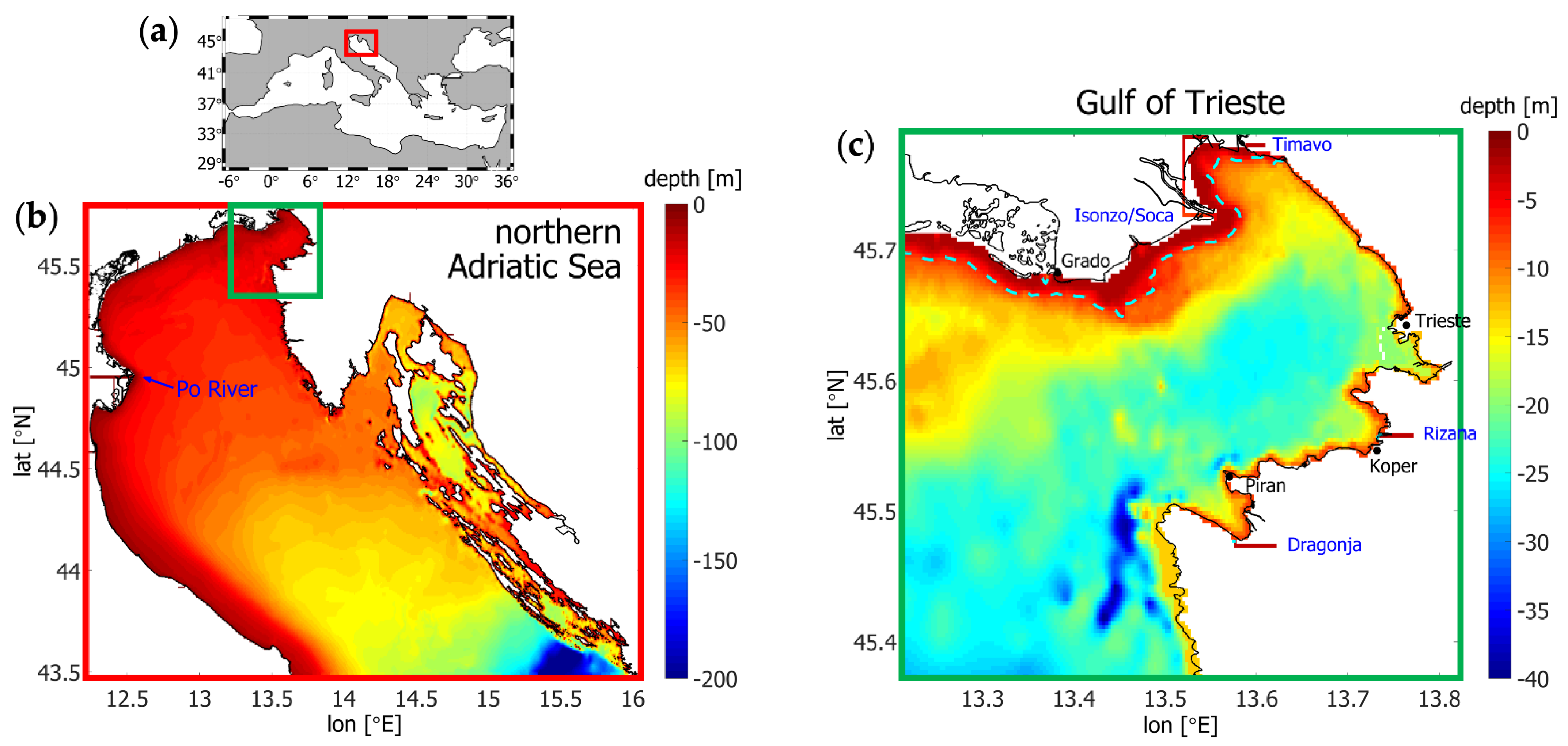The image is a scientifically generated weather graphic depicting bathymetric data of the North Adriatic Sea and the Gulf of Trieste, divided into three sections labeled as images A, B, and C. 

- **Image A** occupies the top left corner and shows a white map against a gray background, outlined with blue and white dotted lines. It highlights a region within a red box, featuring latitude and longitude markings ranging from 29°N to 44°N and -6°E to 30°E, respectively.

- **Image B**, located in the bottom left corner within a red-border box, illustrates the Northern Adriatic Sea. The map within this image uses a color gradient from dark red to dark blue to depict varying water depths, labeled from 0 meters (dark red) to -200 meters (dark blue). Key landmarks such as the Po River are marked, and longitude ranges from 12.5°E to 16°E and latitude from 43.5°N to 45.5°N.

- **Image C**, positioned in the right corner within a green-bordered box, details the Gulf of Trieste. Similar color coding from dark red to dark blue indicates depths from 0 meters to -40 meters, with longitude spanning from 13.3°E to 13.8°E and latitude from 45.4°N to 45.7°N. Prominent labels include Timago, Isonzo, Soca, Gredo, Trieste, and Rizana.

The overall visual emphasizes shallower waters near the coast progressing to deeper waters further out, represented through a spectrum of colors transitioning from red to blue.